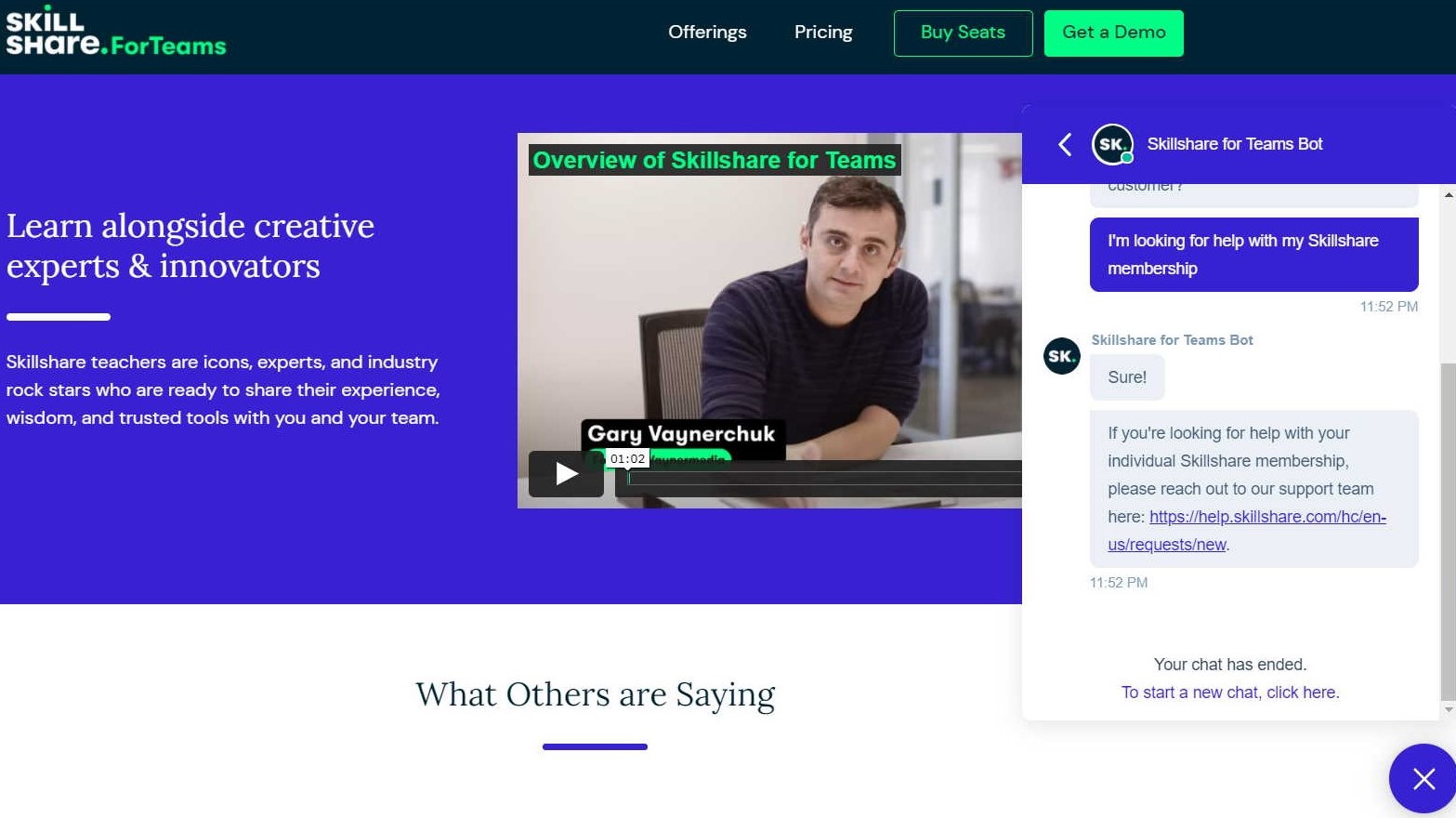The homepage of Skillshare features a top border approximately one inch in height, filled with a very dark blue color, particularly concentrated in the top left corner. Prominently displayed in bold white text, the logo reads "skill" atop "share", with a small green dot above the "i". Adjacent to "share", there is another green dot, followed by the text "for teams" in green. Towards the middle, small white lettering lists "offerings" and "price". A green-bordered tab labeled "buy seats" appears in green, while a separate green tab with the inscription "get a demo" stands out against the dark blue background. 

Below this header, the background transitions into a deep blue hue. On the left side, roughly midway down the page, large white lettering states "learn alongside creative", with "experts, innovators" below. A thick white line separates the word "experts", followed by three lines of additional information.

To the right, there is an image of a man seated at a desk, equipped with a play button in the lower-left corner. The backdrop consists of a white wall and desk, and the man, sporting a black shirt and black hair, is the focal point. Above and to the left of him, a black bar contains the text "overview of Skillshare for teams" in green. His name, "Gary Vaynerchuk", is written just above the play button, slightly to the right.

On the right-hand side of the page, a blue tab holds a circular black emblem with "SK" in it, followed by white text that reads "Skillshare for teams". Beneath it, there's a blue rectangle icon with a speech bubble, indicating there are two lines of dialogue and a date in the bottom right. The next response from Skillshare says "sure", and following that is a full paragraph of text. At the bottom, it states "your chat has ended. To start a new chat, click here."

Adjacent to the picture, under a white background, is the section "what others are saying" in black text. A blue line runs along the bottom right corner, culminating in a blue circle with a white "X".